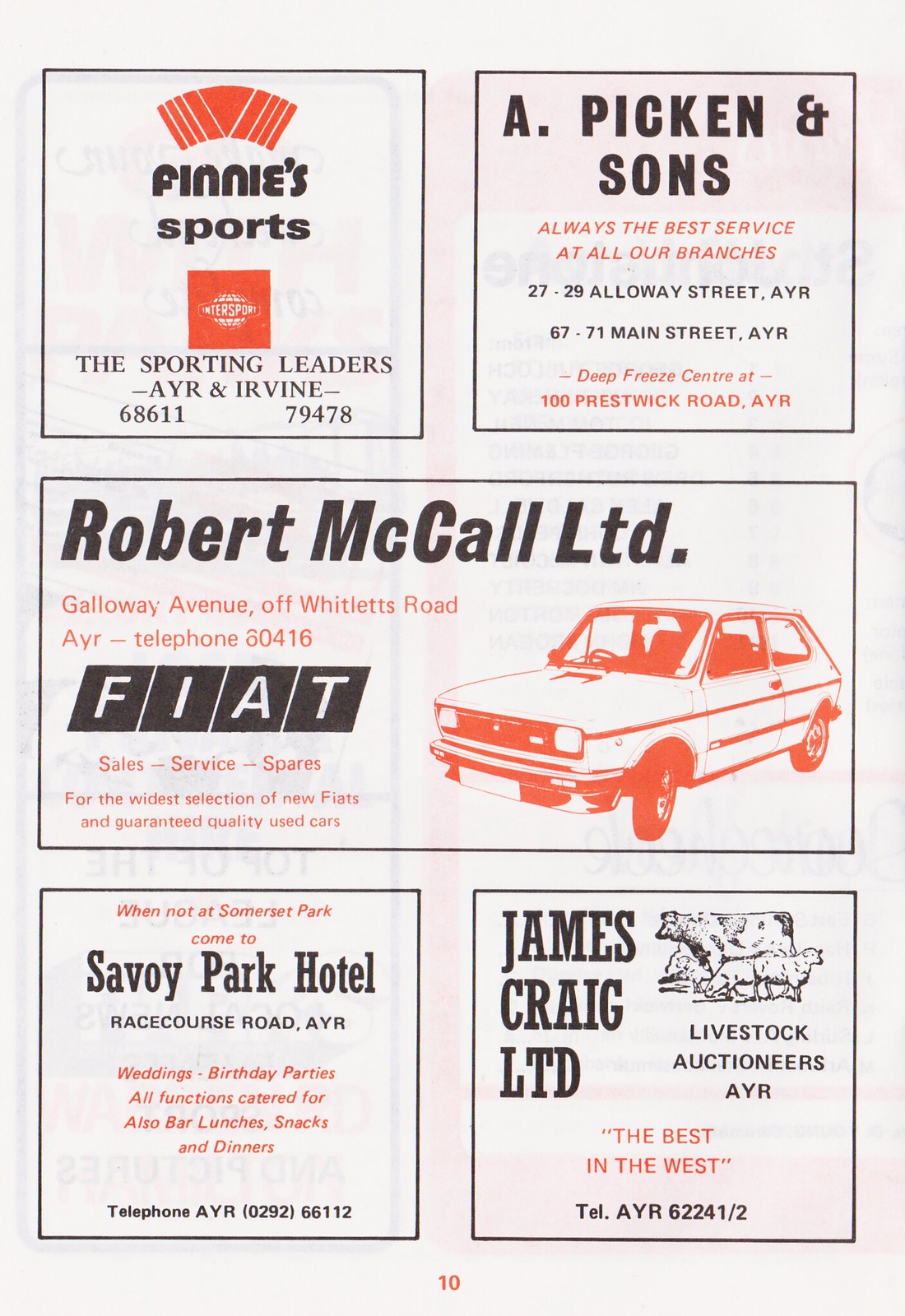The image is an advertisement layout designed to promote various businesses, presumably appearing on the back of a publication. The background is an off-white sheet, possibly resembling old paper or a placemat you'd find in a restaurant, filled with distinct sections for each business.

At the top left corner is an orange square promoting "Finney's Sports" with the tagline "These Sporting Leaders" and their contact number, Irvine 6861179478, written beneath. Adjacent to it on the top right is an ad for "A. Pickin & Sons" featuring an orange line of text that states, "Always the best service at all our branches."

The central rectangle is dedicated to "Robert McCall, LTD," a company specializing in Fiat service, sales, and spares. A red sketch of a Fiat car is prominently displayed on the right side of the rectangle.

In the bottom left corner, there's a square ad for "Savory Park Hotel" located at Racecourse Road in AYR. Finally, the bottom right corner contains an ad for "James Craig, LTD," Livestock Auctioneers in AYR, with a small piece of livestock clip art, and the phrase "The best in the West."

The entire layout is neat and well-spaced, dominated by white, black, and orange colors, and marked with the number 10 at the bottom, indicating its placement on page 10 in the publication.